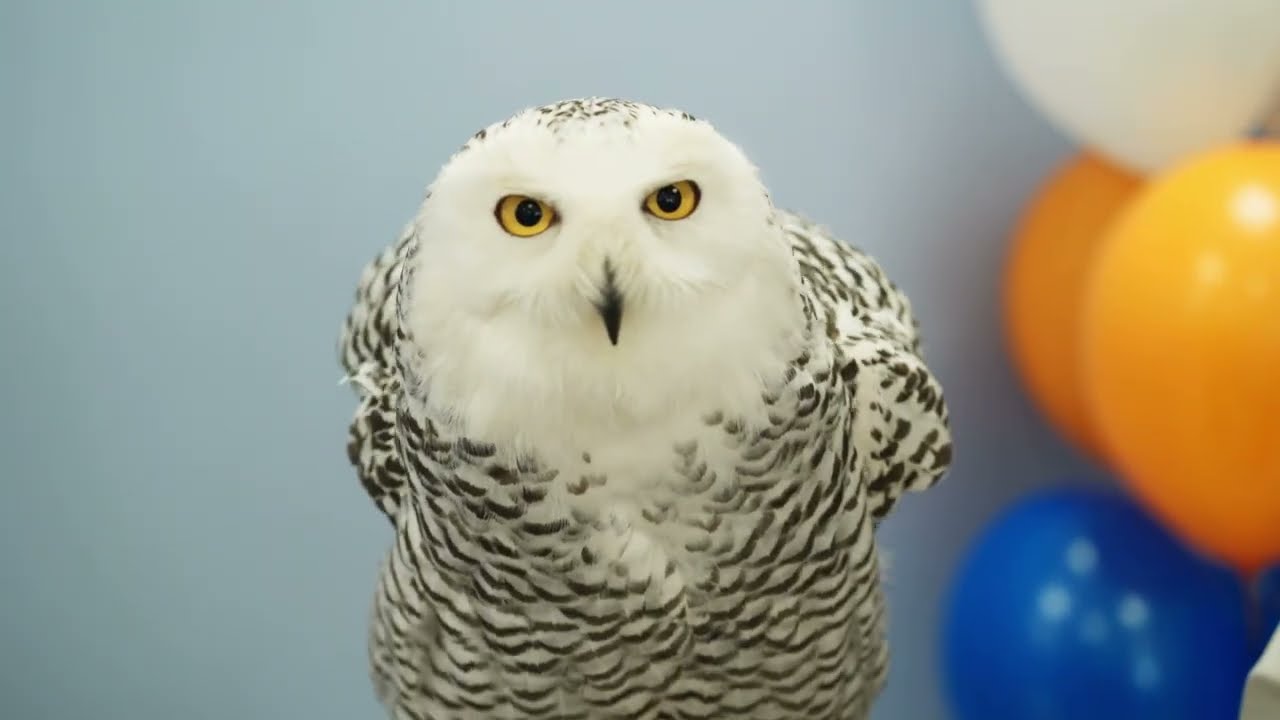In the image, a live owl is prominently displayed in the center, staring intently toward the camera. The owl's head is mostly white with small black spots at the top, and it has striking yellow eyes and a black beak. Its fluffy, black and white feathers cover its body and wings, which are tucked behind its back, giving it a slightly hunched appearance. In the background to the right, there are four balloons: the bottom one is blue, the two middle balloons are orange, and the top balloon is white. The balloons reflect light against a pale blue wall, adding a subtle brightness to the scene. The owl appears still, almost motionless, as it gazes forward.